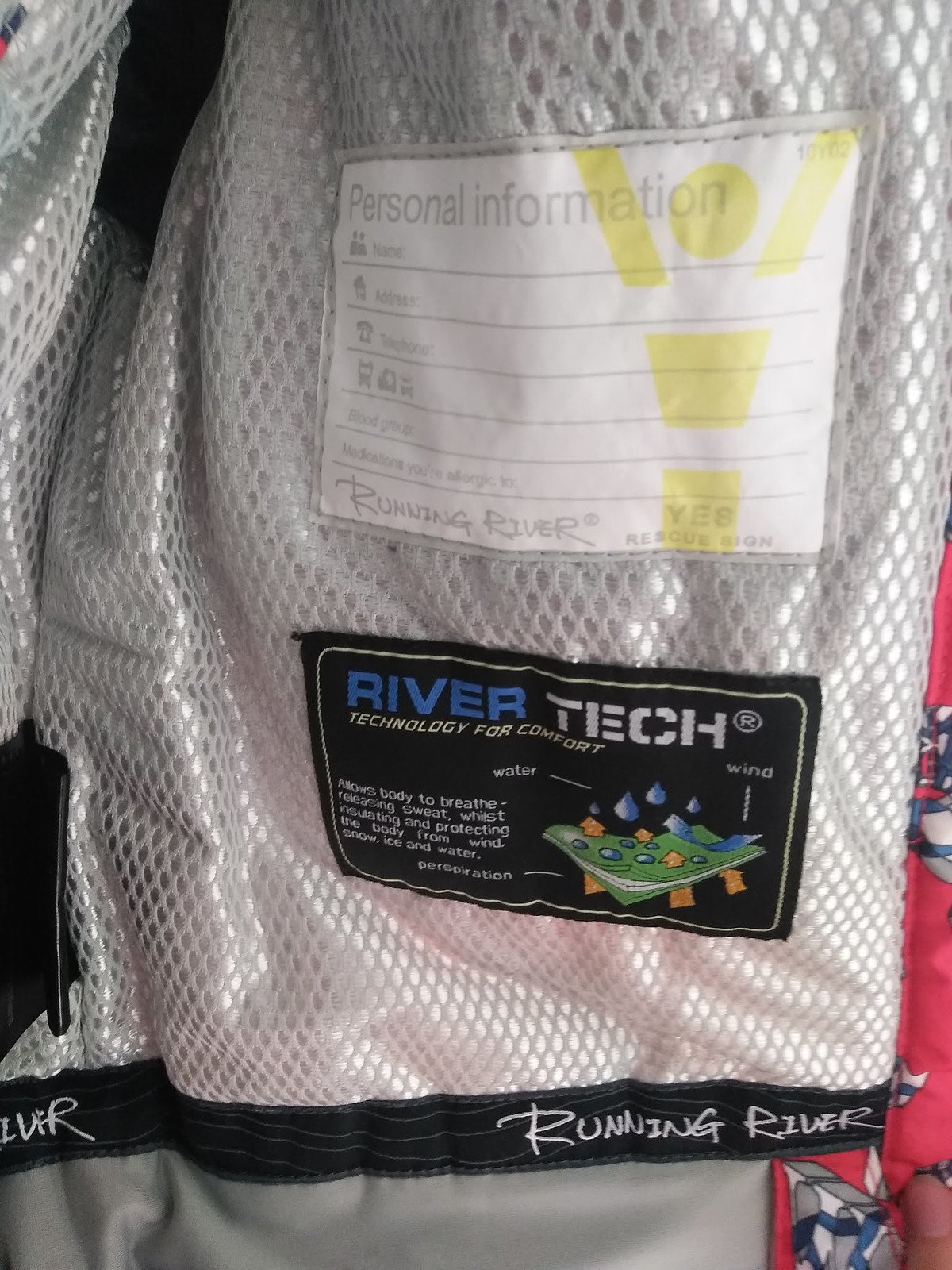The image depicts the interior of a high-tech fitness garment, possibly designed for athletic activities or protective sports like football. The material appears to be mesh-like with integrated padding for added protection and comfort. There is a section designated for personal information, allowing the user to record their name, address, telephone number, and blood group. At the bottom of this section, the label reads "Reading River." Additionally, another label at the very bottom of the garment says "River Tech - Technology for Comfort," indicating that the garment is engineered to allow the body to breathe and manage sweat efficiently, all while protecting against external elements such as wind, snow, ice, and water.